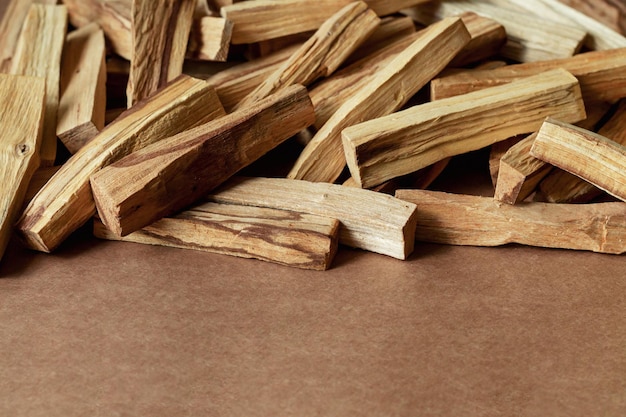This image features a close-up of numerous small wood chips stacked in the upper half of the frame. While some chips appear machine-cut, giving them a uniform size and shape, others look more irregular as if chopped by an axe. The chips vary in color, dominated by light brown hues with occasional dark brown shades. These wood fragments rest on a plain brown surface that could be either the floor or a countertop, blending seamlessly with the wood chips' tones. The composition showcases the textural contrast between the more refined chips and the rustic, hewn pieces, making it look like preparations for kindling, possibly for a hearth or fireplace.